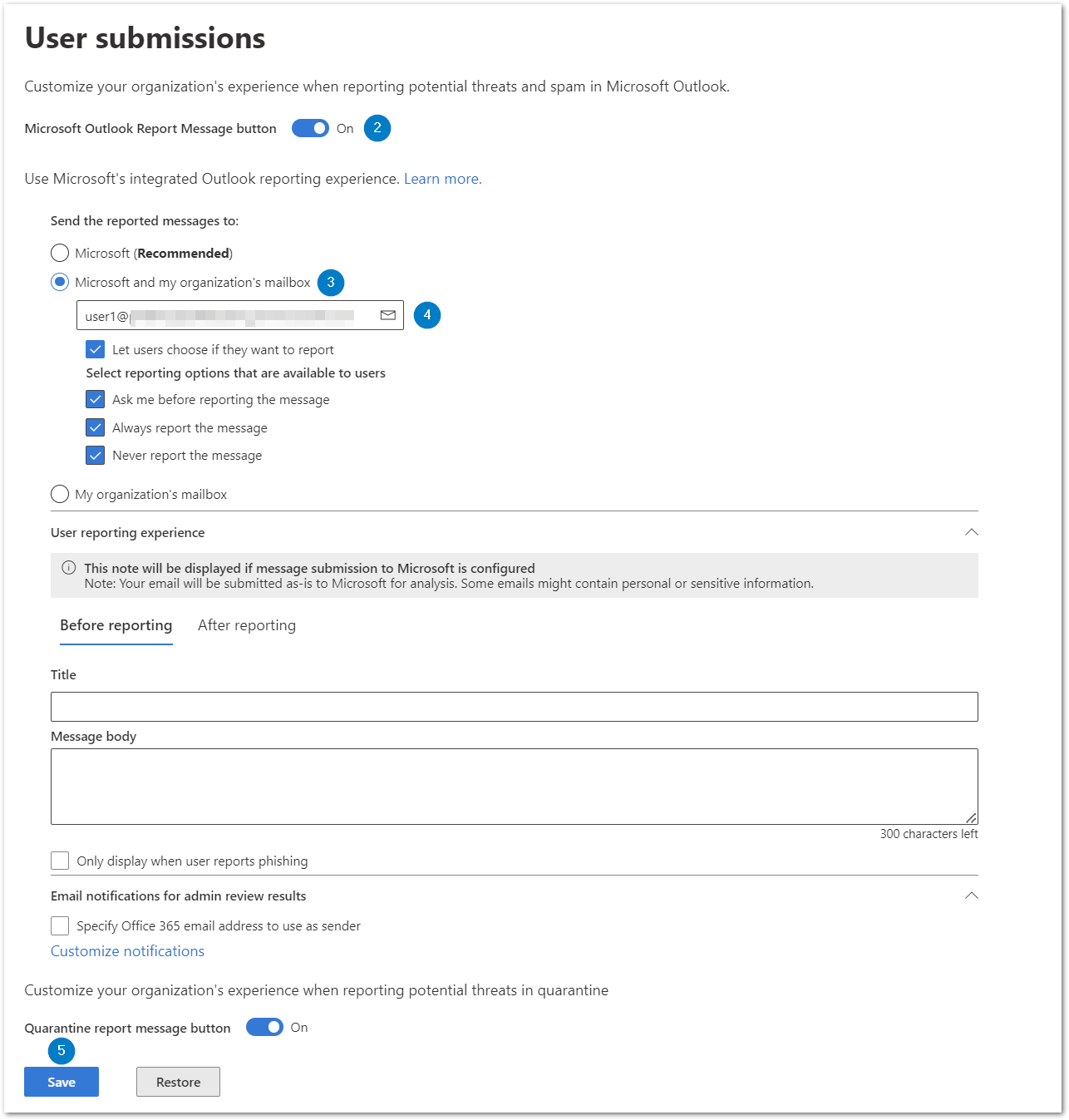**Caption:**

A detailed screenshot of a settings or customization page within Microsoft Outlook, displayed in portrait orientation. The interface features a clean white background bordered by thin gray bars on the left and top, and thicker gray bars on the right and bottom. At the top of the screen, a bold black headline reads "User Submissions," followed by a smaller description: "Customize your organization's experience when reporting potential threats and spam in Microsoft Outlook." 

Beneath this, the text "Microsoft Outlook Report Message Button" appears in black, along with a blue toggle switch indicating that the feature is turned on. A notable blue circle with a white number "2" is displayed, possibly indicating a step or stage number. 

The option "Use Microsoft's Integrated Outlook Reporting Experience" is listed next, followed by instructions: "Send the reported message to," with two radio buttons underneath. The first, labeled "Microsoft recommended," is unselected, while the second option "Microsoft and my organization's mailbox" is selected in blue. There is a grayed-out link below for privacy.

Directly underneath, four checkboxes are all marked in blue. Another radio button is present but not selected. A black divider separates this section from a long horizontal gray box crossing the screen, containing text in black. 

The following segment, headed by the underlined blue text "Before Reporting," highlights input boxes for entering a title and message body, with an edit option available. The layout is structured and user-friendly, offering various customization settings for handling reporting functions within Microsoft Outlook.